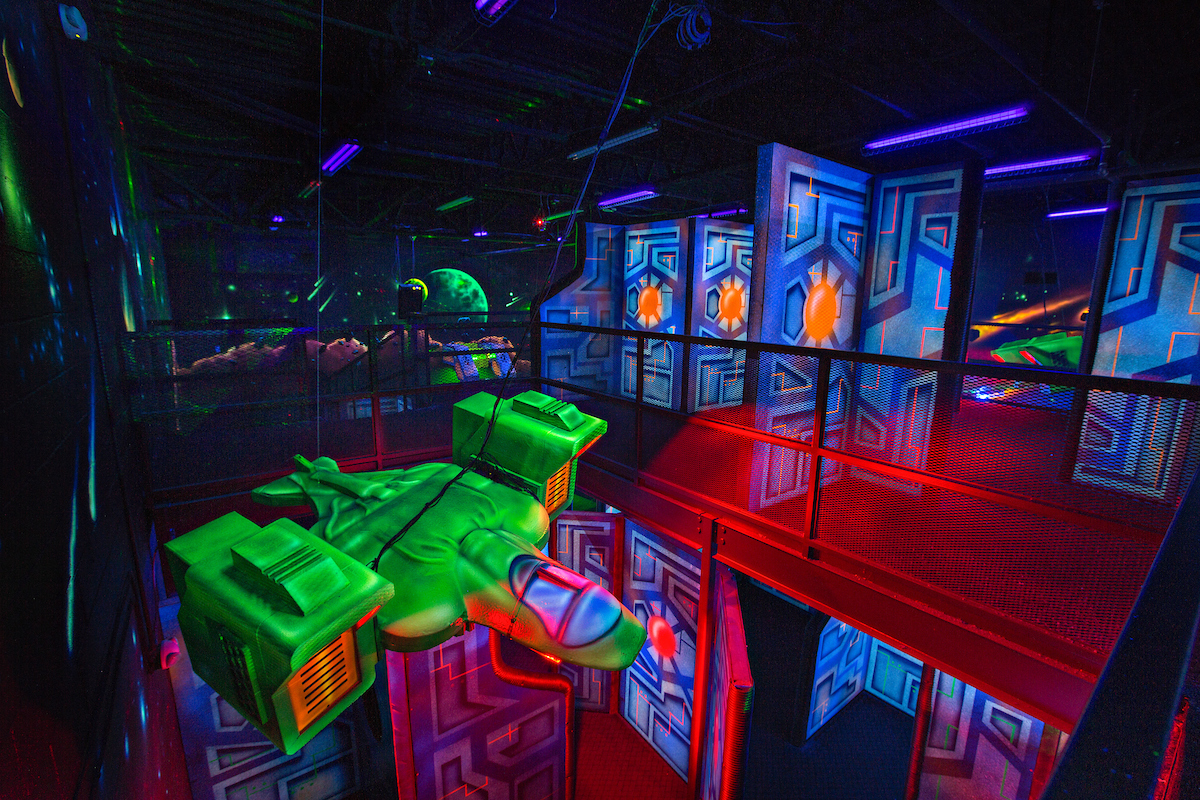The vibrant and neon-drenched scene depicts an indoor game or arcade space, possibly designed for activities like laser tag or children's gatherings. Dominating the foreground is a neon green spaceship, suspended from the ceiling by black cables and sporting box-like wings with golden grates. Below it, the image showcases a labyrinth of blue and gray walls, each adorned with bright orange circles, resembling stylized, cartoonish spaceship doors. The scene is layered, with a metal railing on the second floor offering a view of the bustling space below. In the backdrop, a colorful mural illustrates a cosmic vista with planets, a green neon moon, planetary mountains, rock formations, and green asteroids tumbling down. The entire space glows with a spectrum of neon hues—purples, blues, greens, and reds—adding to its otherworldly charm, while red lighting accentuates lower-level areas, giving the environment a dynamic, multi-dimensional feel. The absence of any textual elements allows the vivid imagery to fully captivate the viewer's imagination.